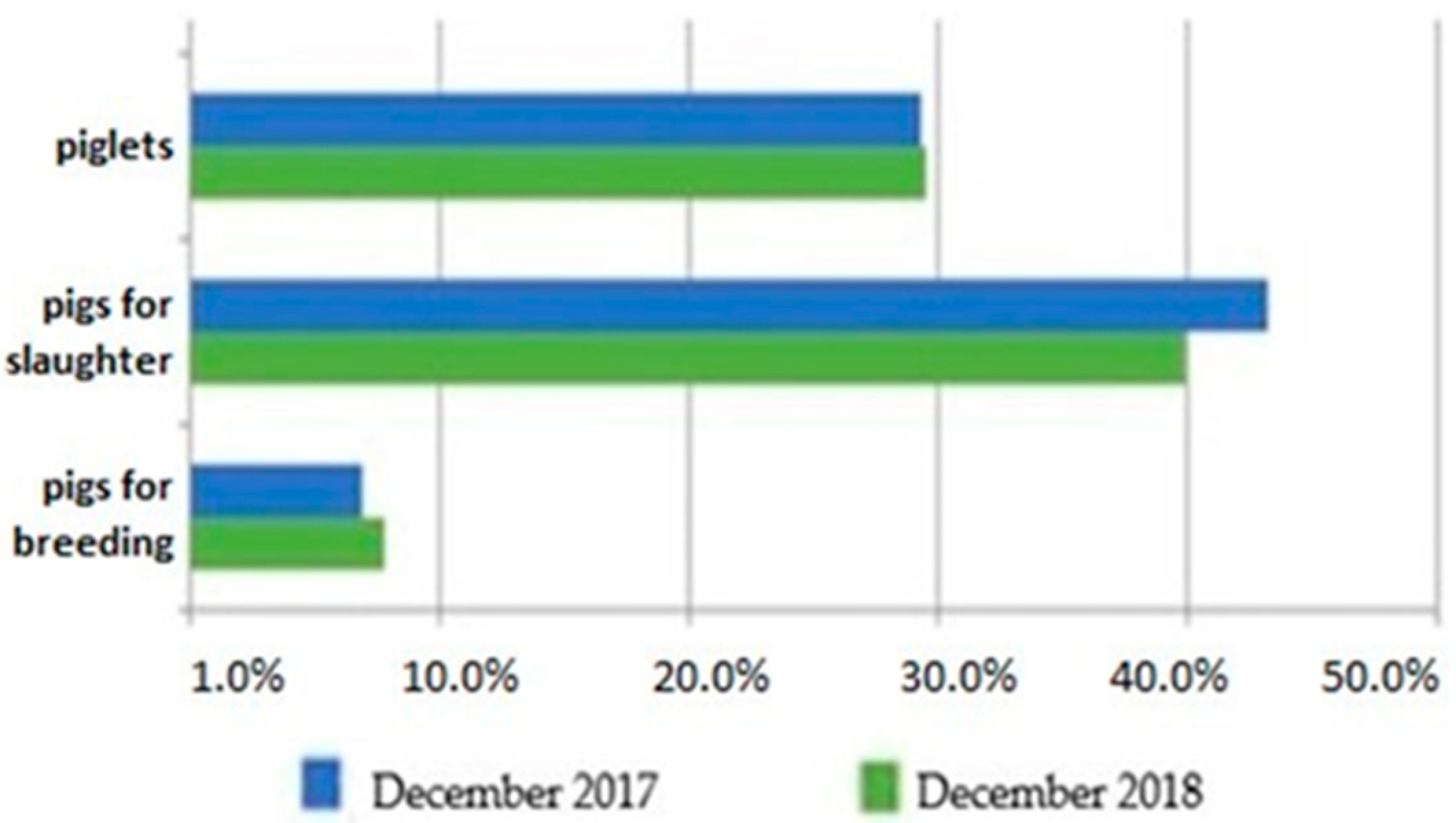The image features a detailed bar chart illustrating the distribution percentages of different categories of pigs along the y-axis. The categories include "Piglets" at the top, followed by "Pigs for Slaughter," and "Pigs for Breeding" at the bottom. The x-axis is labeled with percentage increments, starting from 1.0% and increasing through 10%, 20%, 30%, 40%, and 50%.

At the bottom of the chart, there is a legend indicating that blue bars represent data from December 2017 and green bars correspond to data from December 2018. 

The data depicted in the bar chart shows:
- "Piglets" maintain consistent percentages for both documented years, standing at approximately 30%.
- "Pigs for Slaughter" are represented by a slightly higher percentage in December 2017, around 43%, while in December 2018, the percentage marginally decreases to about 40%.
- "Pigs for Breeding" are shown with a lower presence, about 7% in December 2017 and a slight increase to approximately 8% in December 2018.